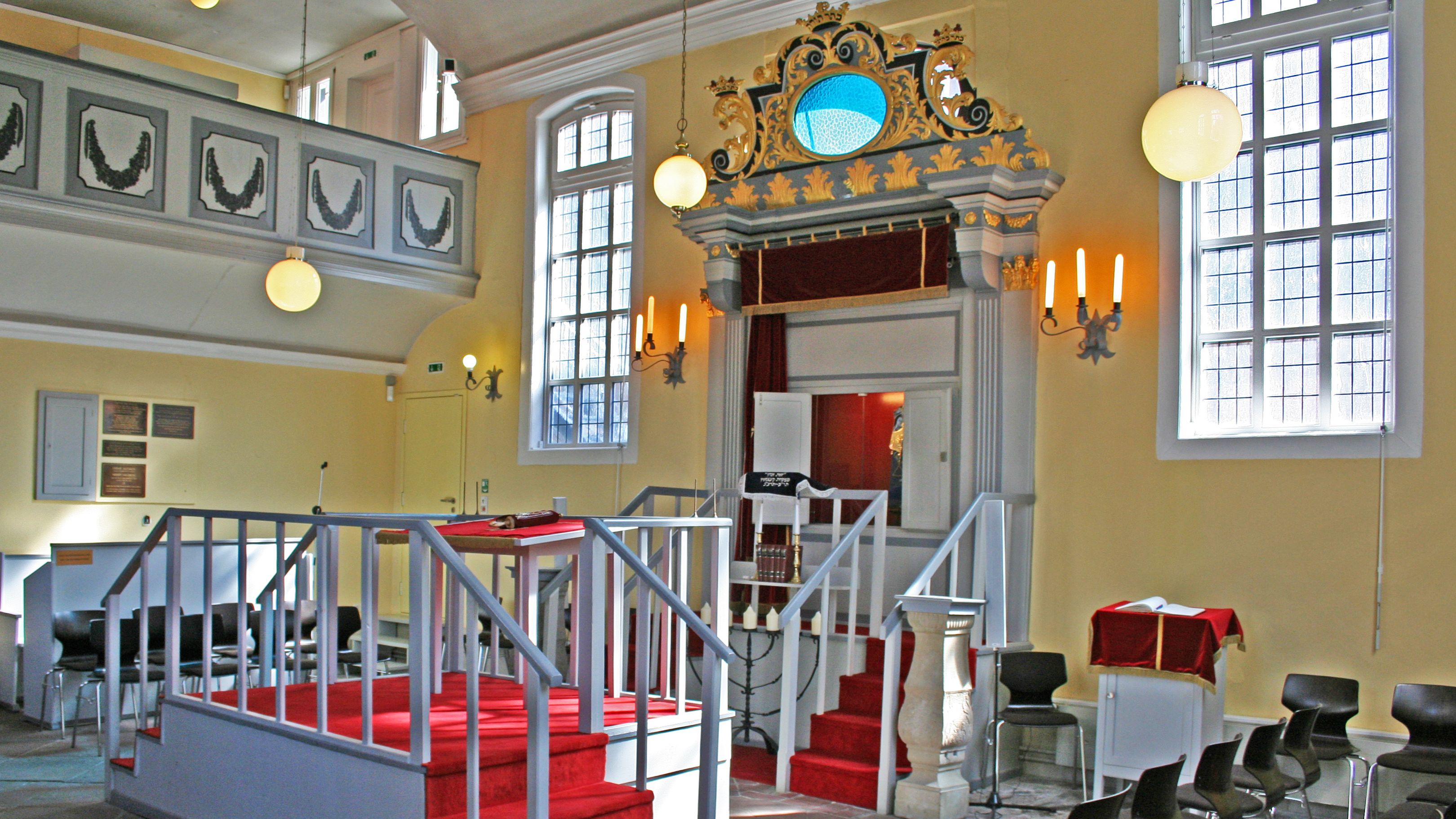The image depicts the interior of a large, ornate room, likely a place of worship or a meeting hall, characterized by its high ceilings and ample natural light. The walls are painted in a yellow-beige hue, complemented by white trim and large windows on both sides of the room. Dominating the center is a raised platform with red carpeting, featuring a white podium and an open book, possibly a Bible. Behind this speaking area, the wall showcases intricate carvings and columns, as well as a golden altar piece with a circular mirror. Flanking the central area are several black plastic chairs, and additional seating is visible in the distance. Round hanging lights and wall-mounted candelabra-style fixtures add to the room's illumination. A well-lit cabinet with decorative detailing at the top can be seen directly behind the podium, reinforcing the space's ornamental aesthetic. A balcony is visible at the upper left, further emphasizing the room's grand scale and intricate design.